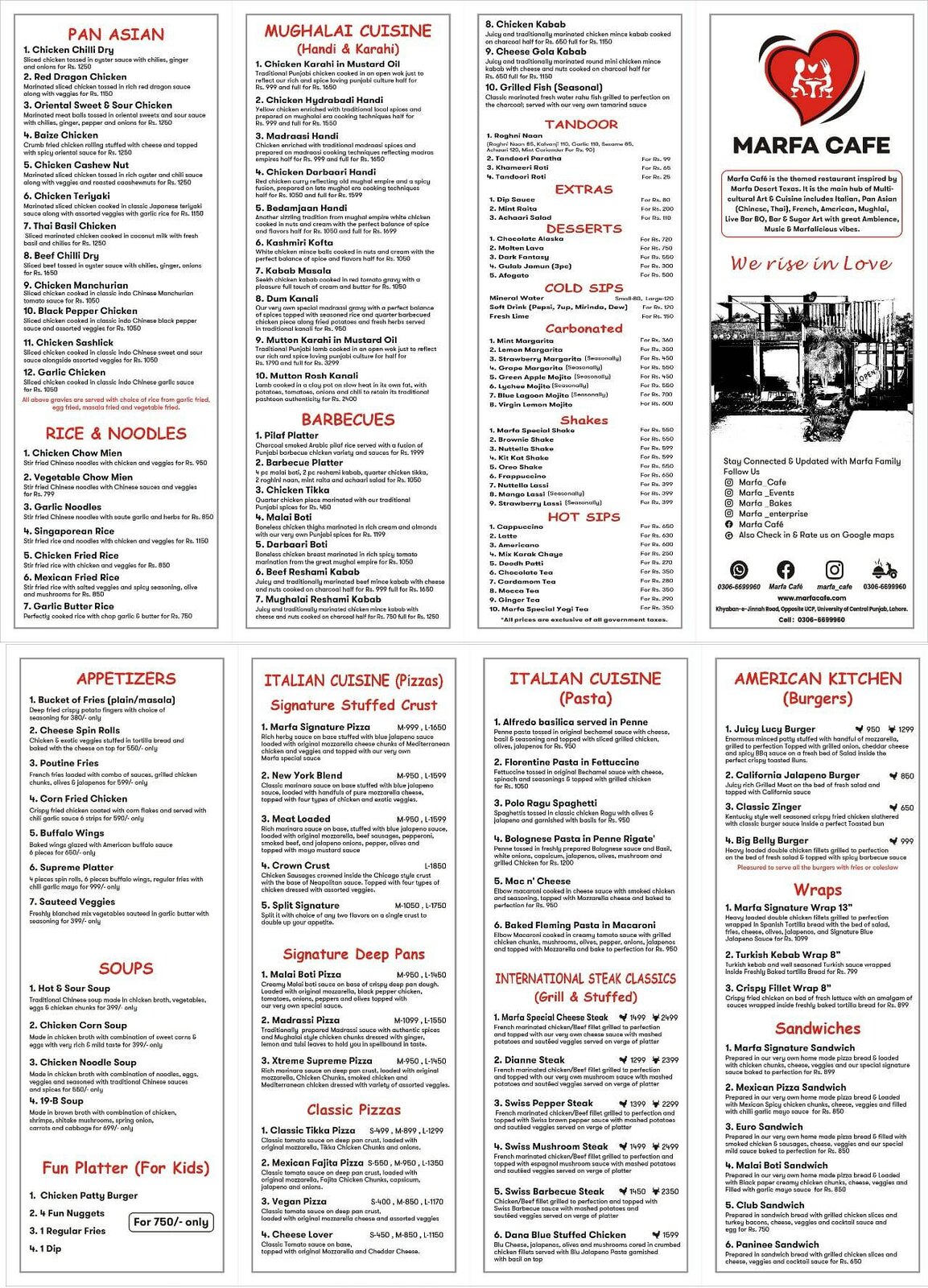This image showcases a comprehensive, unfolded layout of a takeout restaurant menu, presented as if it were a mock-up for print. The menu is divided into two rows, each containing four panels. Here is a detailed description of the contents of each panel:

### Top Row (Left to Right)
1. **First Panel:**
   - Title: "Pan-Asian"
   - Subtitle: "Rice and Noodles"
   - The titles are in bold red font, while the numerous menu options underneath are in black font. There appear to be about 12 items listed under "Pan-Asian" and approximately 7 items under "Rice and Noodles," though the details are too small to read clearly.

2. **Second Panel:**
   - Title: "Mughlai Cuisine"
   - Subtitle: "Barbecues"
   - This panel also features extensive sections under each title, written in smaller black font.

3. **Third Panel:**
   - Multiple Section Titles: "Tandoori," "Extras," "Desserts," "Cold Sips," "Carbonated," "Shakes," and "Hot Sips"
   - This panel is dedicated to a variety of smaller sections, ranging from traditional foods like Tandoori to a selection of beverages.

4. **Fourth Panel:**
   - This panel serves as the front page of the takeout menu.
   - It features the restaurant's name, **Marfa Cafe**, alongside the tagline "We Rise in Love."
   - The panel includes the restaurant's logo, an image of the interior, and various social media icons.

### Bottom Row (Left to Right)
1. **First Panel:**
   - Titles: "Appetizers and Soups"
   - This panel is likely filled with a variety of starter options and different types of soups.

2. **Second Panel:**
   - Titles: "Italian Cuisine," "Signature Deep Pans," "Classic Pizzas"
   - This section focuses on Italian dishes, particularly pizzas prepared in deep pans as well as classic pizza varieties.

3. **Third Panel:**
   - Title: "Italian Cuisine Pastas"
   - Dedicated to a selection of pasta dishes, continuing the Italian theme from the previous panel.

4. **Fourth Panel:**
   - Title: "American Kitchen," "Burgers, Wraps, and Sandwiches"
   - This final panel offers a variety of American-style dishes, including burgers, wraps, and sandwiches.

In summary, the menu is intricately detailed and categorizes a wide range of cuisines, offering an extensive choice to cater to diverse tastes.